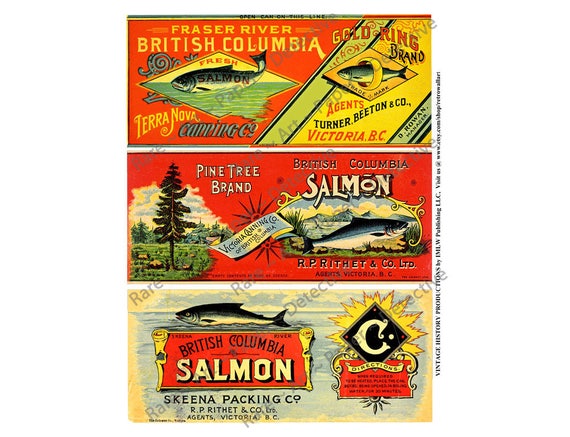The image showcases a vintage advertisement for fresh salmon from British Columbia, divided into three distinct sections. 

At the top of the image, framed in red and yellow hues, the label reads "Fraser River, British Columbia, Fresh Salmon" in yellow font. It also includes "Gold Ring Brand" and mentions the agents "Turner, Beaton & Company, Victoria, BC, Terra Nova." 

The middle section, with a white background, prominently features a pine tree logo on the left and a picture of a salmon to the right. This label reads "Pine Tree Brand, British Columbia Salmon" in bold text.

Finally, the bottom of the image, which has a light blue and yellow background, displays another red banner that says "British Columbia Salmon" in blue and off-white fonts. Accompanying it is an emblem on the right, framed within a letter 'C,' set against the colorful backdrop, completing the advertisement. 

Each section collectively exudes an old-fashioned charm, with recurring themes of British Columbia and fresh salmon vividly depicted.